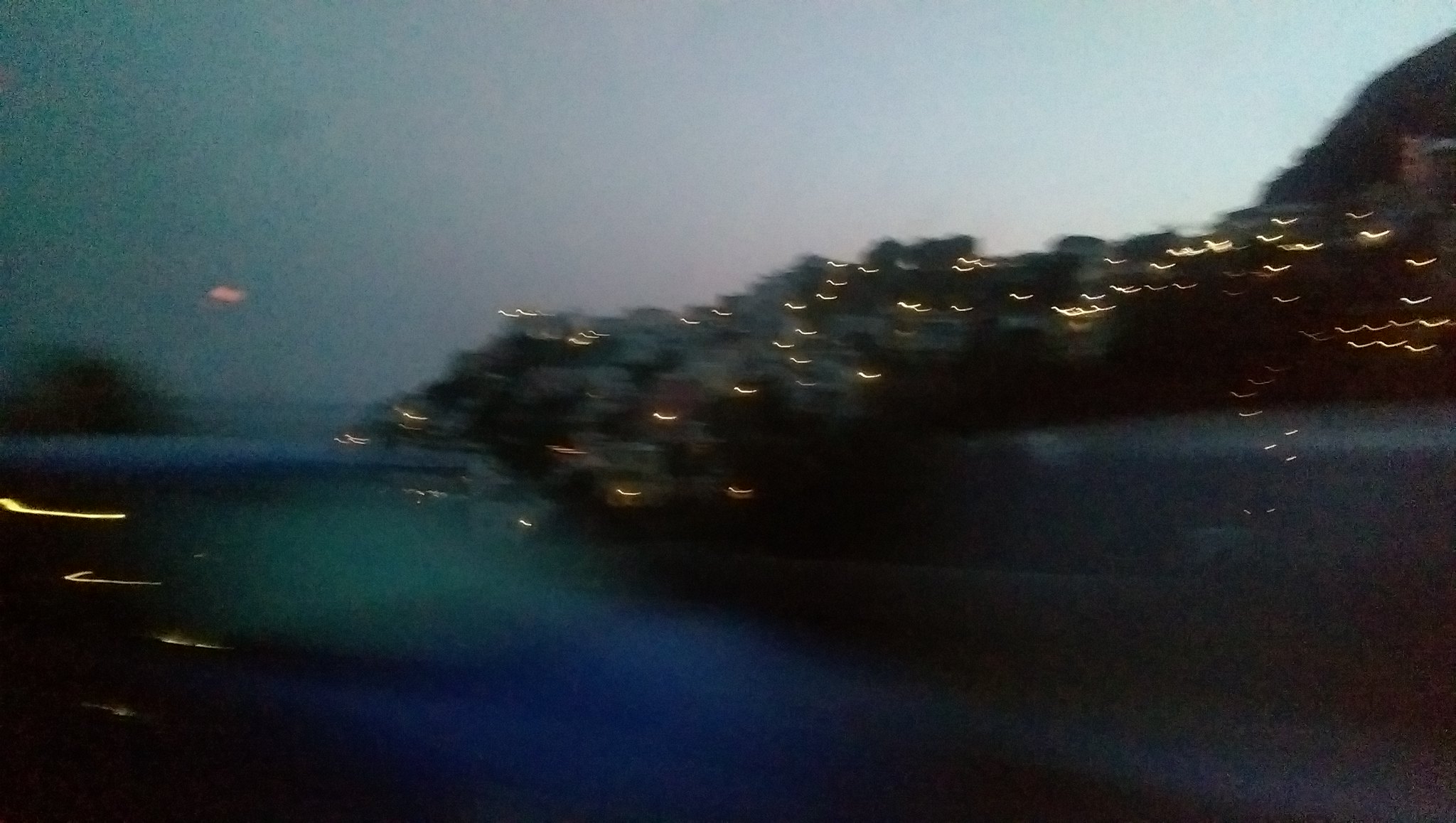The image is a blurry, out-of-focus color photograph capturing an ambiguous outdoor scene. At the top, the sky is visible in various shades of blue, transitioning into pink and light blue, with a dark grayish hue on the left side. In the middle and upper right section, the silhouette of what appears to be a mountain or hill is dotted with numerous small lights, roughly 20 to 30, giving the impression of distant buildings or vegetation. On the left side of the image, there's a bright, glowing area, possibly a cloud or the Sun, surrounded by yellow laser-like lines about two inches wide. The foreground of the photo contains a blurred blue object, possibly a car with light reflecting off its windshield, suggesting movement towards the right. Near the bottom left, there's an indistinct shape that could be an island or part of a vehicle, bordered by greenish-blue water. Parts of the background feature what looks like a cinder block wall with vegetation spilling over it, further adding to the photo's enigmatic quality.